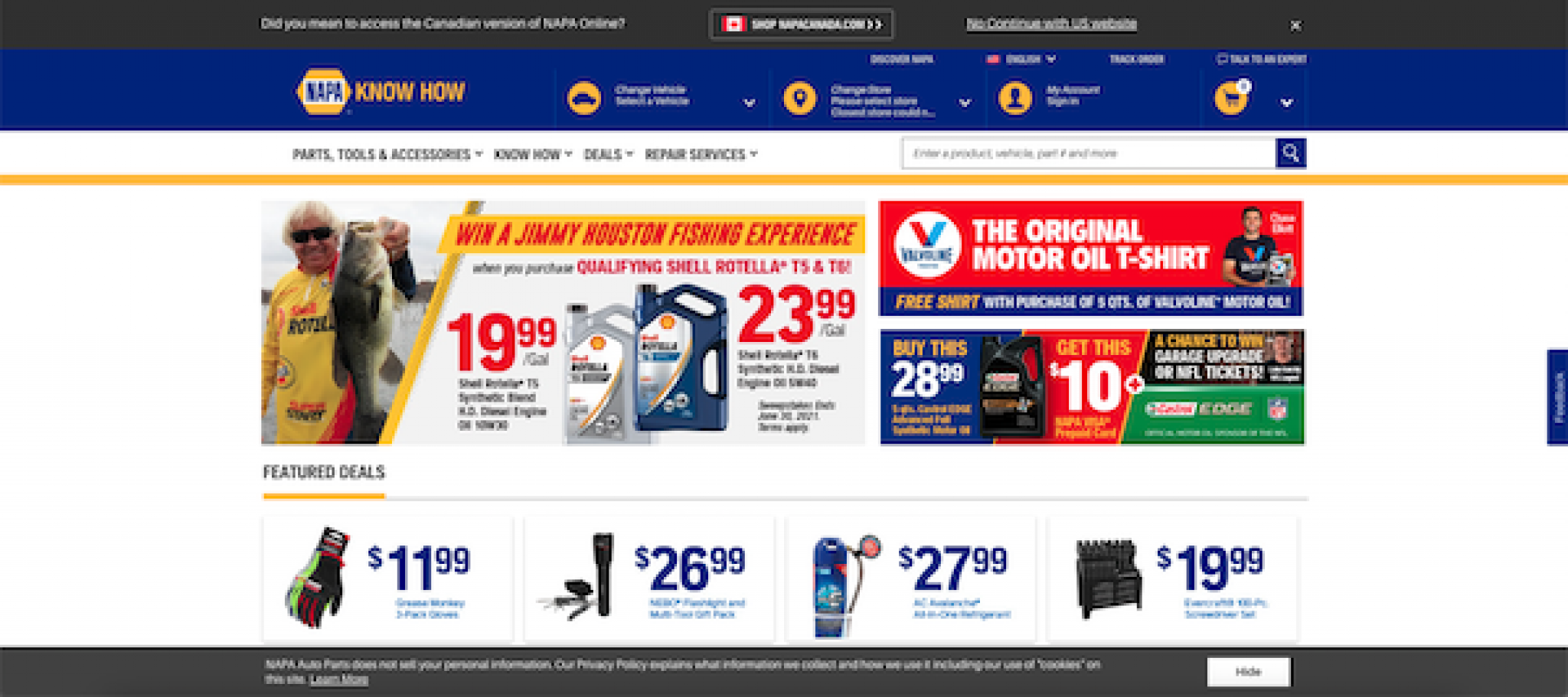The image depicts a web page advertisement for NAPA Auto Parts. The top section of the page is slightly out of focus, but prominently features the NAPA brand tagline "NAPA Know How." The advertisement showcases a variety of auto parts, tools, and accessories as part of their promotional deals and repair services.

A central visual element shows a man with white hair and glasses, wearing a yellow shirt, proudly displaying a large bass fish. This image is associated with a promotional offer to win a fishing experience with Jimmy Houston by purchasing qualifying Shell Rotella ATS products priced at $19.99 and $23.99.

Additionally, the ad highlights a special offer from Valvoline, noting that customers can receive a free Valvoline "The Original Motor Oil" t-shirt with the purchase of a 5-quart bottle of Valvoline motor oil. The motor oil retails for $28.99, and there's an added incentive to get a $10 discount, as well as a chance to win either a garage upgrade or NFL tickets.

Towards the bottom of the ad, several featured deals are listed, including:
- $11.99 for gloves
- $26.99 for a flashlight
- $27.99 for an unspecified item (the image of which is blurred)
- $19.99 for drill bits

The very bottom of the page contains small, unreadable white text, alongside a white button labeled "Hide."